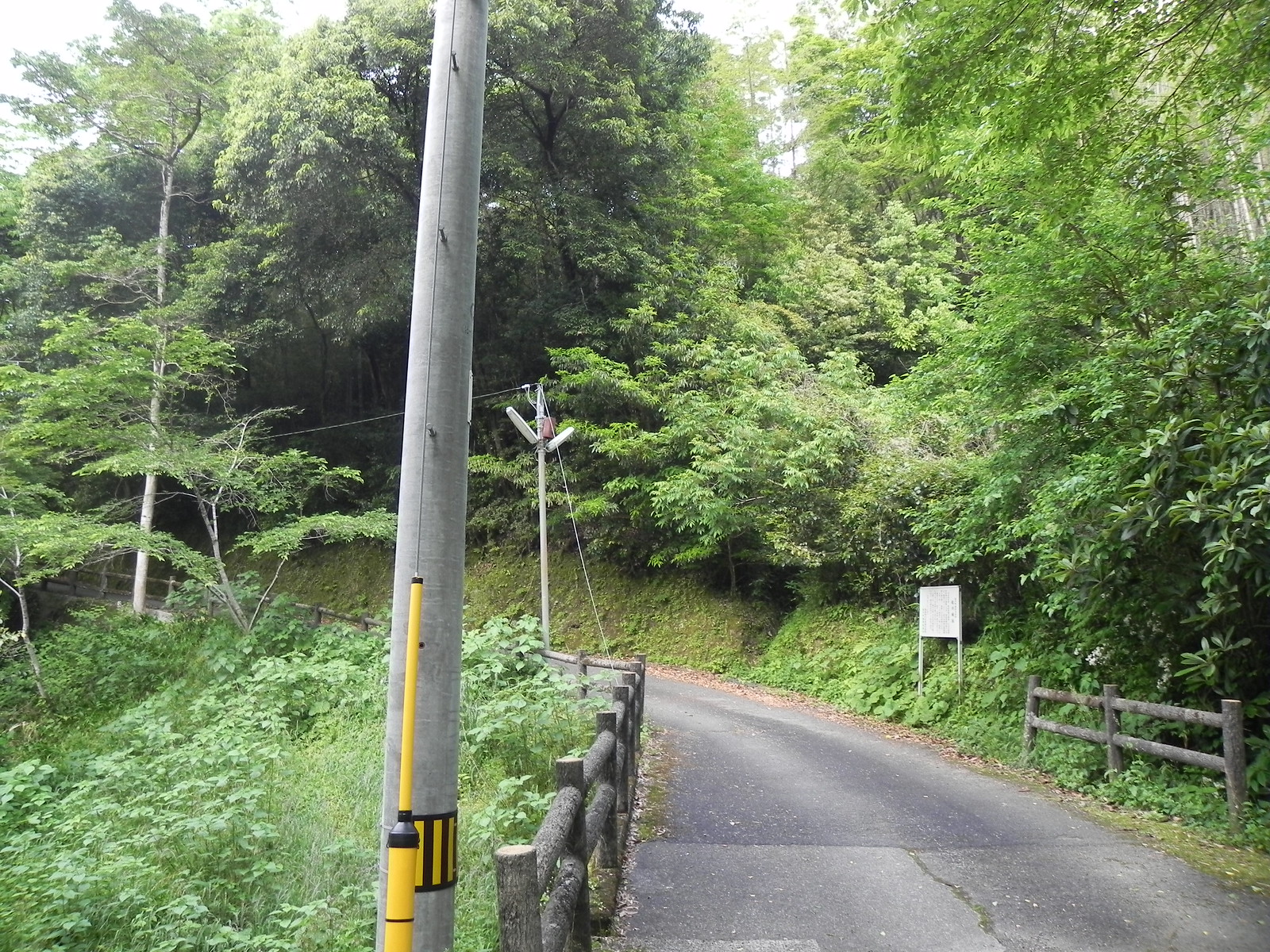The image depicts a peaceful, narrow, curved trail, likely intended for biking or walking, situated in a wooded and hilly area. The trail is flanked by dense foliage and tall trees on the right side. On the left edge, there is a wooden post fence, while on the right side, a shorter section of fence suggests a steep drop-off, indicative of safety measures. 

Stringing alongside the trail are utility poles supporting power lines, some of which are fitted with street lamps. A standout detail is a yellow support string attached to one of the poles. A sign is visible on the right, although its message is indiscernible due to its small size. The trail itself is made of blacktop and curves gently to the left. 

The scene is accentuated by the tranquil colors of green from the lush vegetation, yellow from the support string and possibly the trail markers, and the muted gray of the pathway and poles. The overall atmosphere hints at a scenic mountain road, reminiscent of those found in Japan or Taiwan, providing a serene countryside experience, though it would be advisable to avoid walking there alone at night.